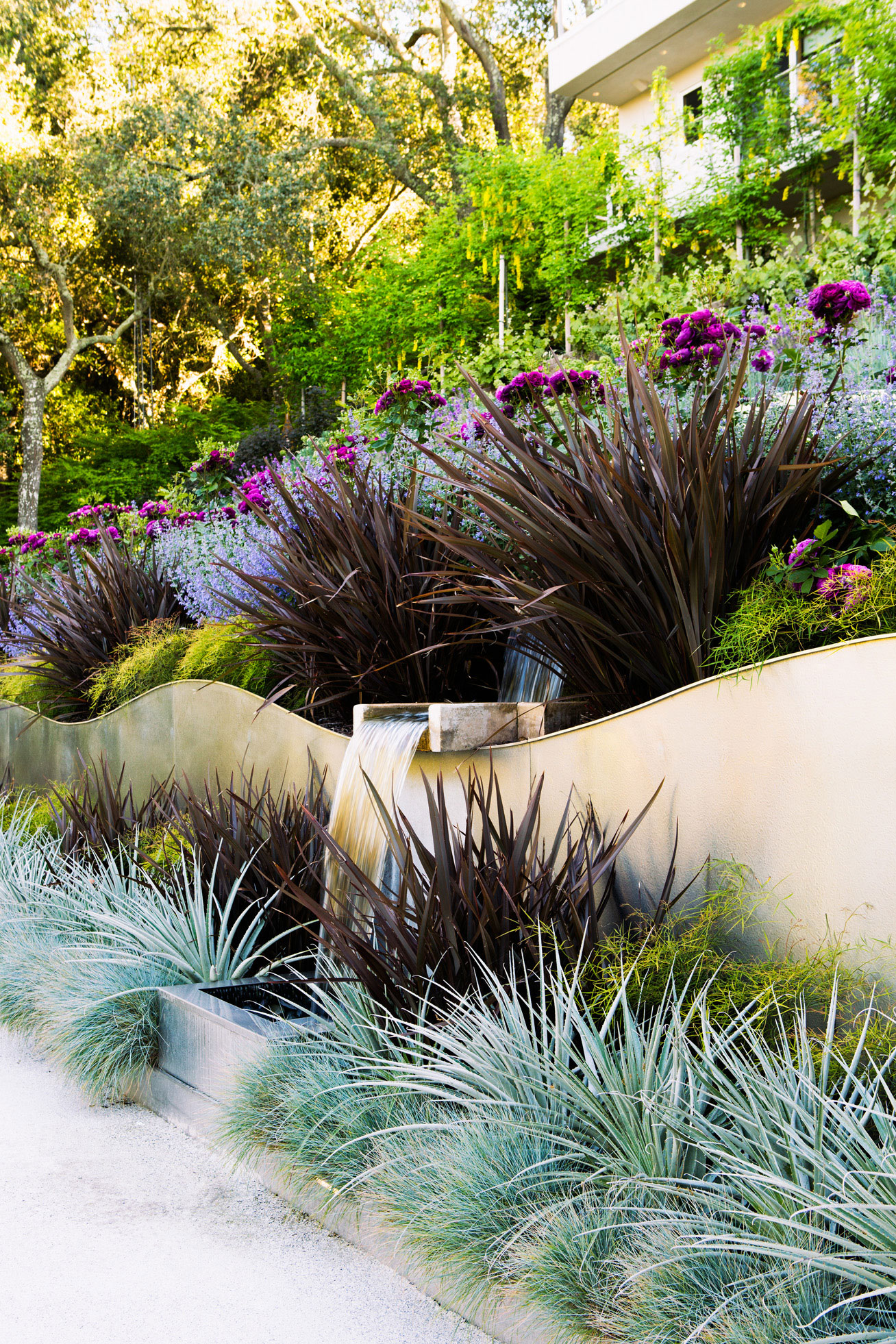The photograph captures an outdoor daytime scene focused on a vibrant and steep hillside landscape, dominated by a meticulously crafted retaining wall made of sloped tan cement, situated at the bottom of the slope. This wall features a central rectangular box from which a gentle waterfall cascades into a catch basin below. In front of this retaining wall lies a diverse array of flora, including spear-shaped grasses in hues of light blue, maroon, and green. Above the wall, the hillside is adorned with a profusion of plant life, highlighted by spiky dark green plants with large clusters of bright purple flowers. Among these, there are also aloe-shaped plants and other desert greenery interspersed with lighter greens and occasional white florals.

The photograph further extends upwards and to the right, revealing a house perched atop the hill, partially obscured by dense vegetation. The structure, some parts seemingly on stilts, is flanked by tall, mossy trees that add to the scene’s lushness. The upper left corner of the image shows more dense trees, while leafy vines drape over a fence, adding a charming, slightly wild touch to this multi-layered snapshot of natural beauty and human architecture.